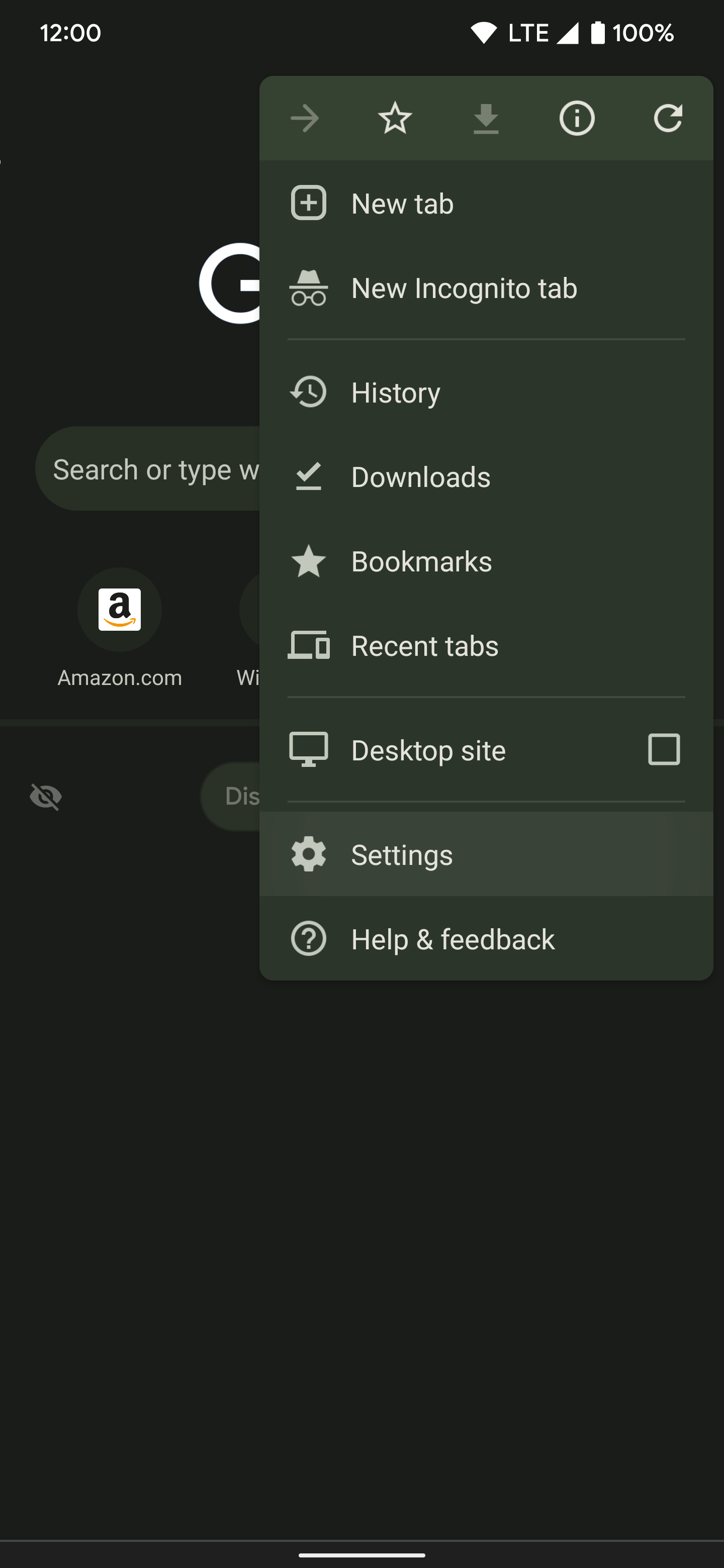The image shows a smartphone screen with several visible details. The phone is operating on an LTE network and shows a full battery charge at 100%. The time displayed is 12:00 PM. The screen itself is primarily black with a prominent white "G" in the center. A popup menu is also present on the screen, displaying several icons and options.

The options listed in the popup menu include:
- New Tab
- New Incognito Tab
- History
- Downloads
- Bookmarks
- Recent Tabs
- Desktop Site

Each option is accompanied by its respective icon, with "Settings" represented by a gear icon and "Help & Feedback" represented by a circle with a question mark.

Behind this popup, the main screen shows a partially visible search bar where the text is cut off, displaying only "W." Leading to a snippet of an Amazon link showing the Amazon logo ("A" with an arrow) and part of the URL "amazon.com." There’s also a gray icon with a line through it and a partially obscured bubble with "DIS" in black, indicating a possible disrupted network or service.

The image encapsulates a typical smartphone interface with a focus on web browsing and the settings menu.